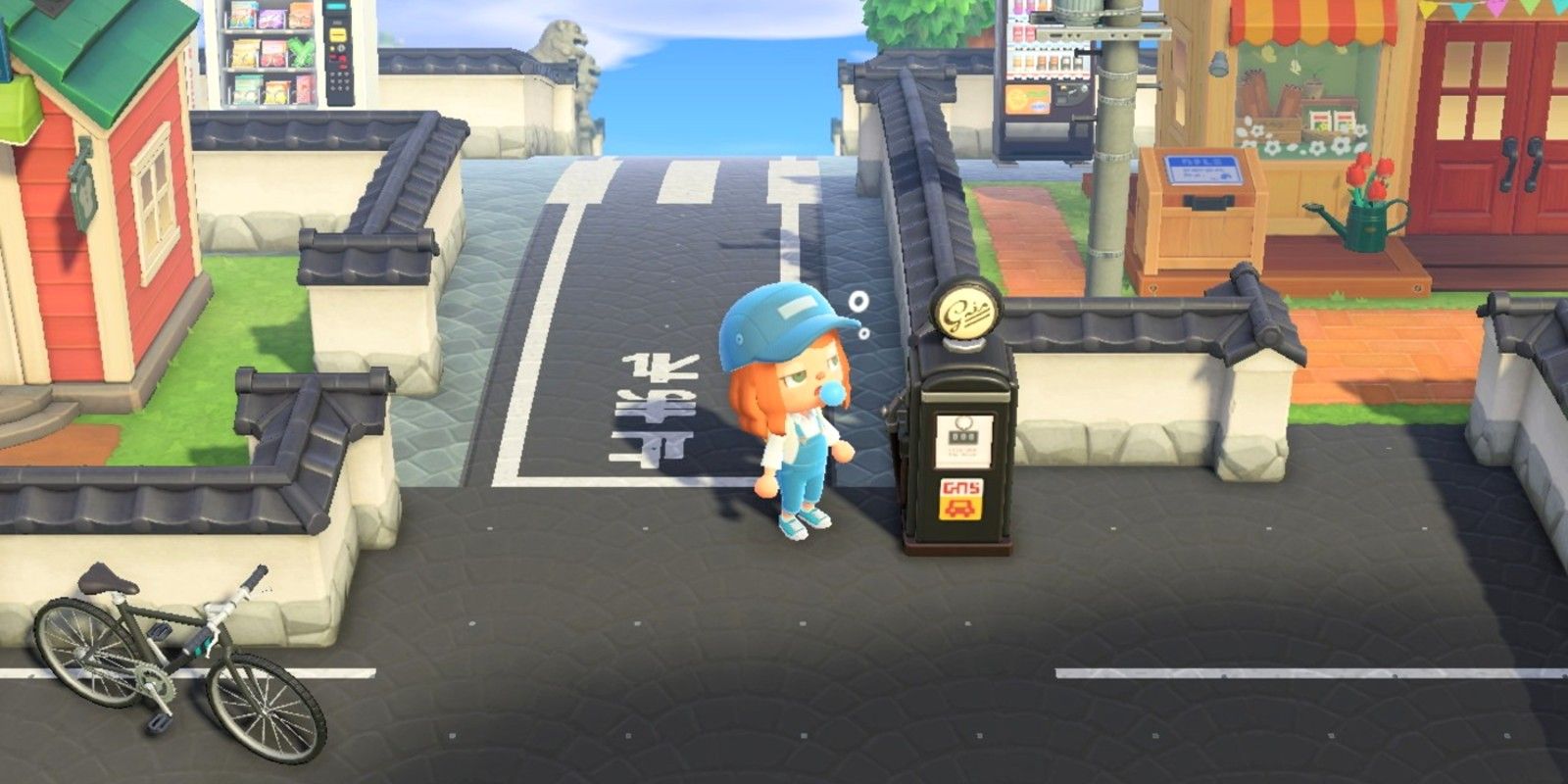In this detailed digital rendering of a vibrant, small Japanese city street, the focal point is a young girl with shoulder-length orange hair, green eyes, and a blue hat. She's dressed in blue overalls, a white shirt, and matching blue and white sneakers. The girl stands centered in the image, blowing a blue bubble next to an old-fashioned black gas pump with the word "gas" displayed on it. Directly in front of her is a street that curves up a gentle hill. The street features a crosswalk with three dashed lines and white-painted Chinese characters. A bike is parked at the bottom left corner, adjacent to a small one-story red house with a green roof and a surrounding fence. To the far right, partially hidden, is a shop or restaurant also enclosed by a fence. The scene captures a mix of colors including black, blue, red, white, green, brown, and hints of yellow. The serene sky overhead is mostly clear with occasional clouds, adding a picturesque backdrop to this charming game world, which appears similar to the aesthetic of a Nintendo Switch game.